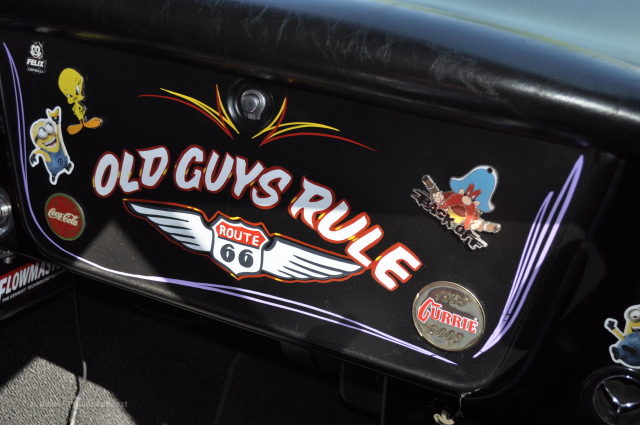This image captures the lower part of a car dashboard, focusing on a glove box adorned with a variety of colorful stickers. Positioned above the foot area of the car, the black glove box features a central lock or button adorned with a small fire design on both the left and right sides. In the middle of the glove box, large white all-caps text with a red outline reads "OLD GUYS RULE." Just beneath this, there's a Route 66 emblem flanked by wings.

The front of the glove box is decorated with several stickers. On the top left corner is Felix the Cat, with Tweety Bird pinned just below. Directly under these is a Coca-Cola logo, accompanied by a small Minion sticker. On the far right, there’s Yosemite Sam from Looney Tunes brandishing his guns with a "BACK OFF" text beside him. Additionally, a smaller circular logo bearing the text "Curie" (C-U-R-R-I-E) is also present on the right-hand side.